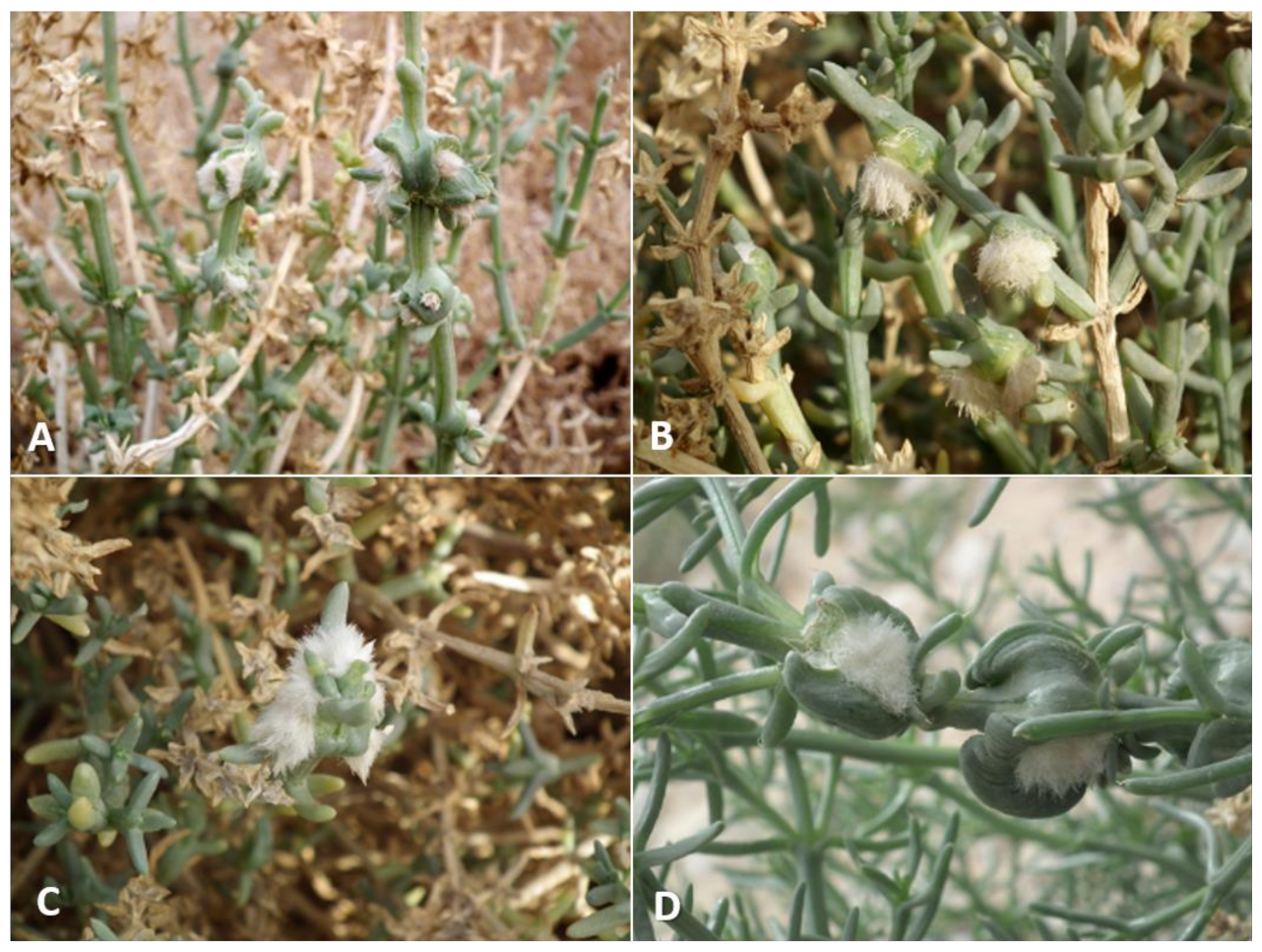This image is a compilation of four scientific close-up photographs labeled A, B, C, and D, each depicting a different stage of plant growth, possibly from a botanical study or database. Image A features green upright stems with small buds and fuzzy, white flowers that have not yet fully opened, set against a dry, brown landscape. Image B shows smaller green plants with more developed, slightly opened buds revealing white, fluffy floral structures. The background is creamy or yellow at the bottom. Image C offers a closer view, highlighting the larger, more detailed white flowers with a cotton-like texture, set against a similar brownish backdrop. Finally, Image D provides a very close view of green stems where multiple stages of the flowering process are visible; the buds are significantly more open, revealing their fluffy, white interiors and giving the impression of cotton balls. The images collectively highlight the plant's growth stages and the development of its distinctive white, fluffy flowers, which may suggest it is a cotton plant or something similar.